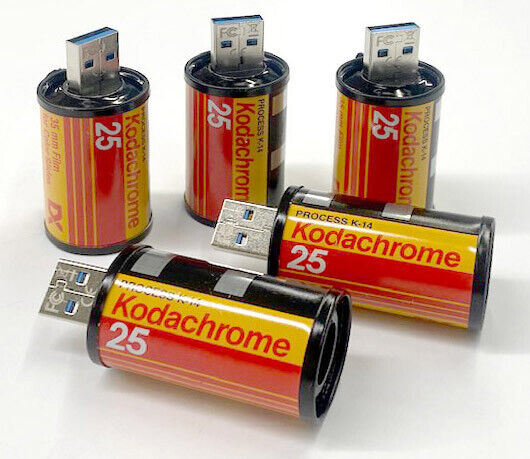The image depicts a collection of five USB sticks designed to resemble vintage film canisters used in cameras from the 1920s and 1930s, where images were burned directly onto the film. These USB sticks, however, are modern storage devices, likely created by a camera brand as a nod to the classic era of photography. Three of the USB sticks are standing upright while two are lying on their sides. The canisters come in blue, yellow, and red, with labels that read "Process K-14" and "Code DACHROME25," adding to their retro aesthetic. This unique design cleverly blends nostalgia with modern technology and serves as an effective marketing strategy for the camera company.